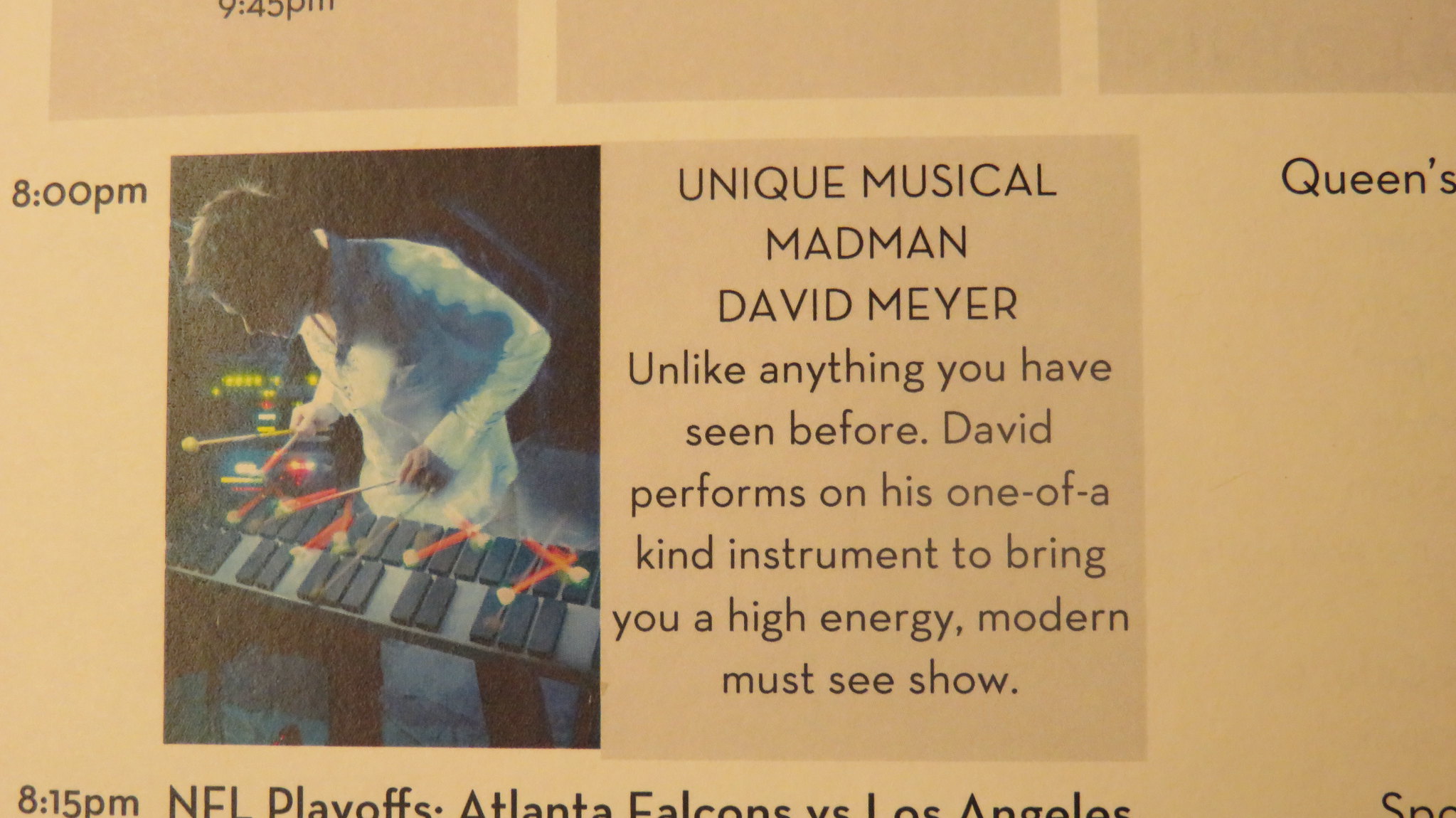The image is an advertisement featuring a Caucasian man, David Meyer, who is prominently displayed playing the xylophone. He is wearing a white long-sleeved shirt and is bent over the instrument, actively striking it with mallets; multiple images of the mallets show movement as they come down on the xylophone keys. To the left of his image, the text "8 o'clock P.M." is clearly visible. Adjacent to the man, bold text declares, "Unique Musical Madman David Meyer," followed by a description: "Unlike anything you've seen before, David performs on his one-of-a-kind instrument to bring you a high-energy, modern, must-see show." Further information is provided beneath this, stating "8:15 P.M. NFL Playoffs Atlanta Falcons versus Los Angeles," though part of this text is cut off. The main color scheme of the advertisement includes black text on a light beige background.